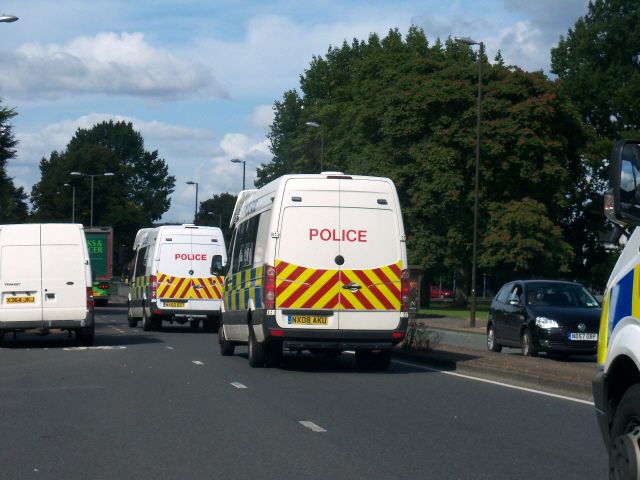This outdoor scene captures a bustling four-lane roadway under a light blue daytime sky speckled with fluffy white clouds. Prominent in the image are three large, boxy police vans, all white with black mirrors and windows. The back of each van displays the word "POLICE" in bold red lettering, accompanied by a striking pattern of alternating yellow and red rectangles. Along the sides, a checkerboard pattern of yellow and blue squares adds to their distinguishing features. The police vans dominate the foreground, while a black VW sedan can be seen coming from the opposite direction. The road is well-defined with white lines marking the lanes and sides. Surrounding this scene, tall, bushy green trees provide a lush backdrop, complemented by numerous tall lampposts scattered along the street. Additionally, there is mention of a green truck ahead and another truck following, underscoring the busy nature of the road where traffic appears to have come to a halt, perhaps due to the police activity. The vehicles’ yellow-backed license plates indicate that the scene is likely set in a foreign country outside of the U.S.